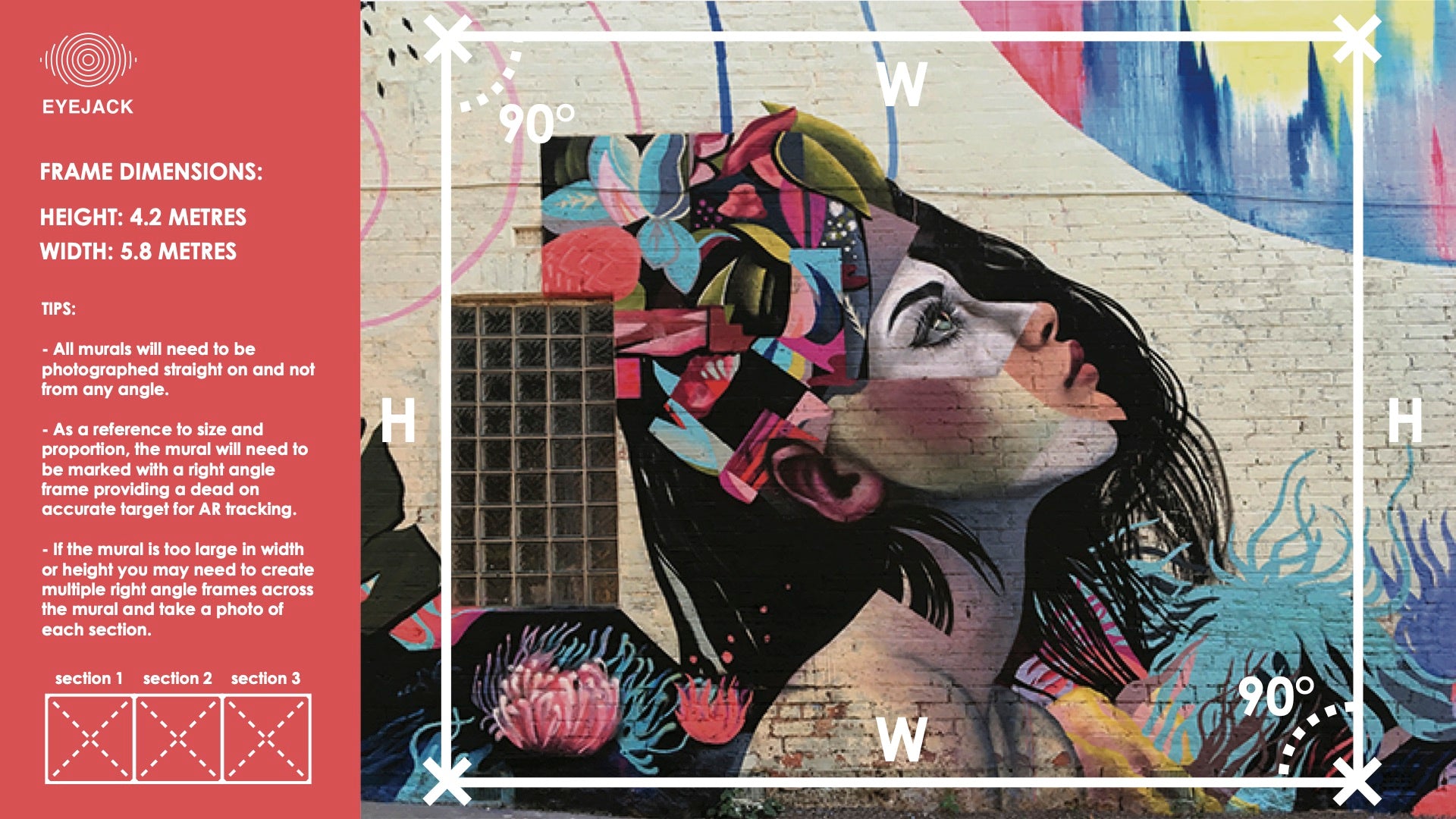The image depicts a detailed mural on the side of a white brick building, featuring a stylized woman with long dark hair and a traditional headdress adorned with flowers, fruits, and various pieces of fabric, possibly indicative of South American or African heritage. She gazes upwards towards the right, towards the bottom corner of a circular object in vibrant yellows, reds, and blues that might represent the Sun or a cityscape. Surrounding her are additional floral designs. On the left side of the image, informational text provides specifics about photographing murals for AR tracking, including dimensions (4.2 meters in height and 5.8 meters in width), and tips for ensuring accurate capture, such as taking photos straight on and possibly using multiple right angle frames for larger murals. The text includes the acronym "IJAC," suggesting it may be related to the entity providing these guidelines.